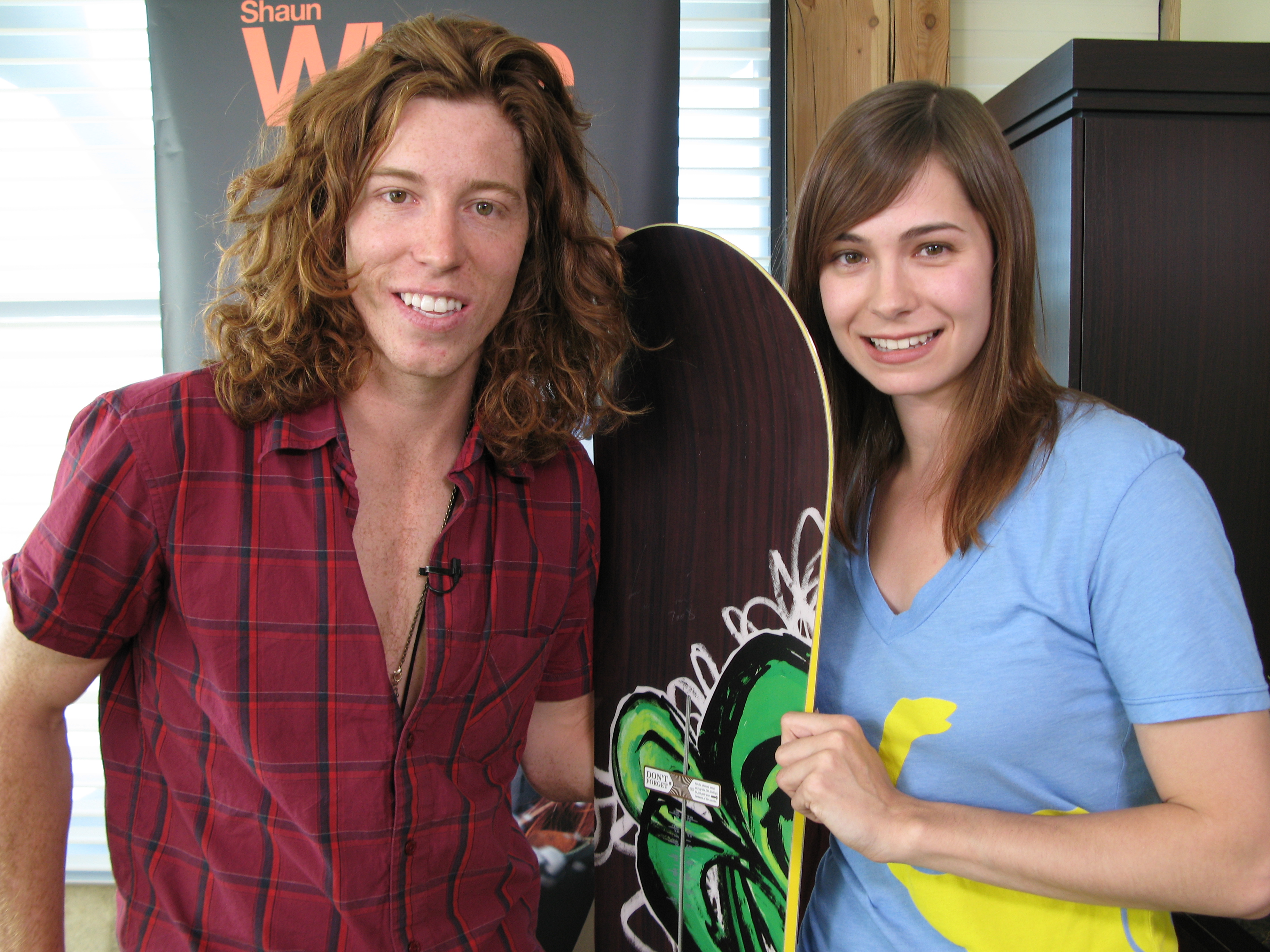The photo features renowned snowboarder Shaun White, wearing a red plaid shirt with the top buttons unbuttoned to reveal a gold necklace beneath. He has a small microphone pinned to his shirt. His long, curly brown hair falls to his shoulders. Shaun stands beside a smiling woman with long brown hair, wearing a blue and yellow T-shirt. Between them, she holds a distinctive snowboard with brown edges and a green, black, and white graffiti-style design in the center. The backdrop includes a partially visible black poster with “Shaun White” written on it, a window, and a dresser, indicating they are indoors. Their friendly demeanor suggests Shaun is likely meeting with a fan.